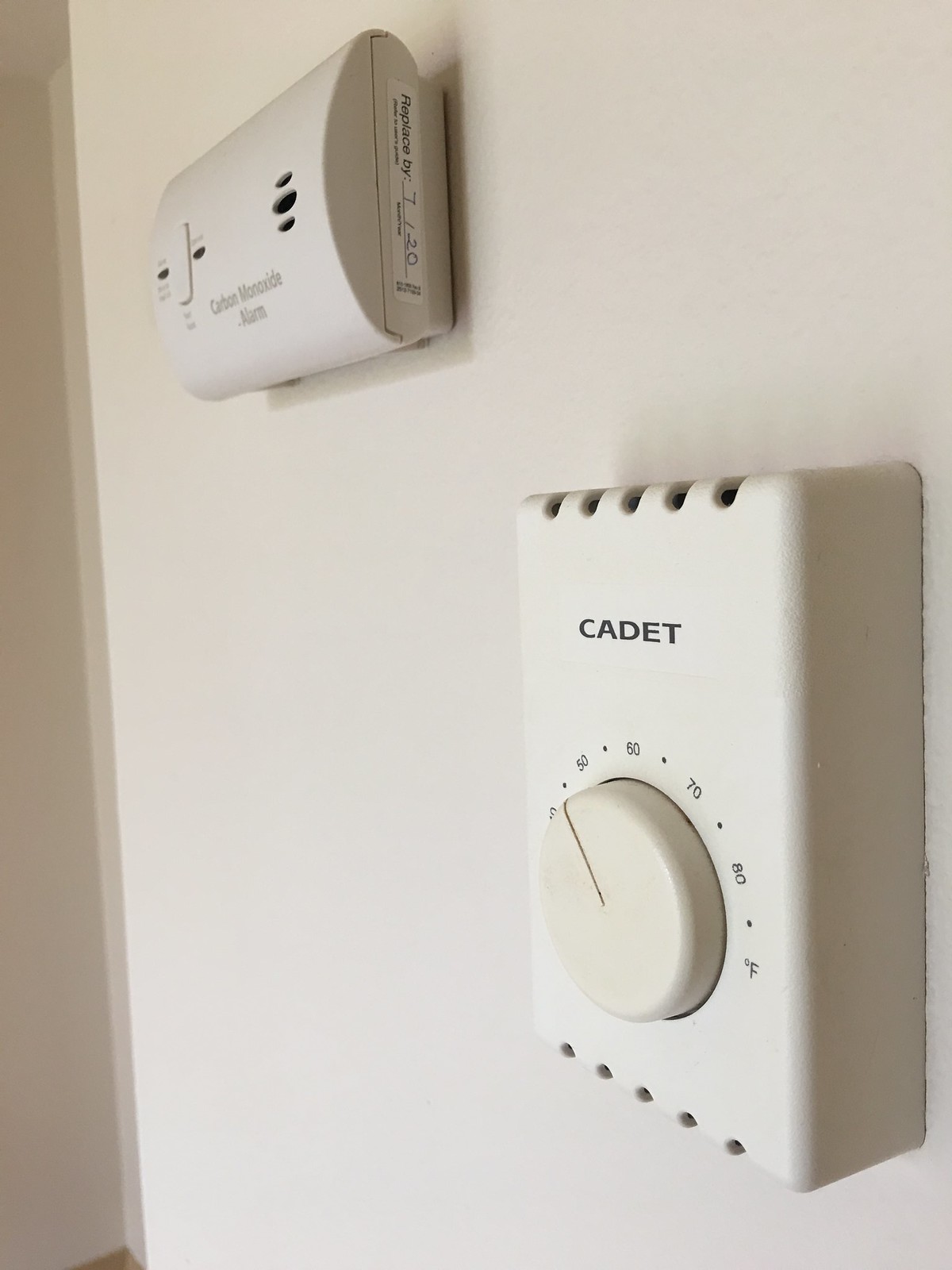This photograph depicts an off-white thermostat and a carbon monoxide alarm mounted on a similarly colored wall. The thermostat, branded "Cadet", is square-shaped with ventilation grilles on the top and bottom. It features a dial that ranges from approximately 40°F to 80°F, currently set to around 51°F or 52°F. The dial has an engraved line indicating the temperature setting.

Beside the thermostat, there is a rectangular carbon monoxide alarm. This device includes three detection holes, a central push button, and two LED indicator lights. The text "Carbon Monoxide Alarm" is prominently displayed on its surface. A tag on the side of the alarm indicates a replacement date of "7/4/20," although the complete date is partially obscured.